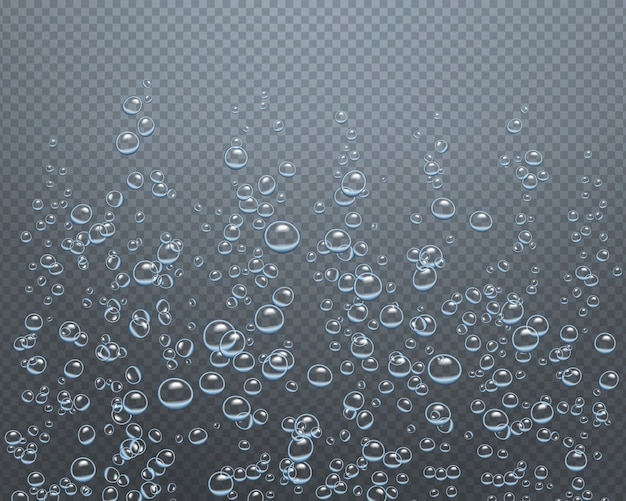This digital artwork features a sea of translucent bubbles ascending from the bottom to about four-fifths of the way up the image. The background is a small-checkered pattern of dark gray and light gray squares, giving it a distinctly digital aesthetic. The bubbles, outlined in a bluish-gray hue, come in various sizes, ranging from very small to quite large, and their distribution varies enough to prevent monotony. Despite their transparent centers, the bubbles are easily distinguishable against the dual-tone checkered backdrop. This image, which appears to be computer-generated and possibly crafted using software like Photoshop, would make a visually arresting background for a computer or phone screen. No text, watermark, or additional elements are present in the artwork.